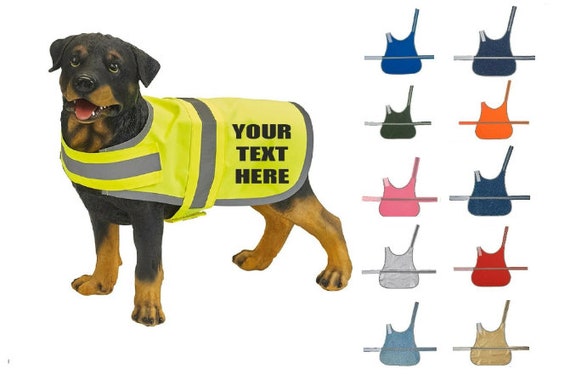This advertisement features a small, black and tan dog, possibly a Rottweiler puppy, wearing a fluorescent yellow safety vest. The vest, which is designed to be visible at night, covers the dog's main body but leaves its legs exposed, and is fastened with Velcro around the chest and underneath the body. On the rear hip area of the vest, there's customizable text that reads "Your Text Here," indicating a space where a business name or message can be added for advertising purposes while walking the dog.

Next to the dog is a chart displaying 10 different color options for the safety vest. The available colors include blue, light blue, dark blue, brown, tan, pink, orange, red, gray, light gray, and greenish hues. These vests are spread out next to the dog in the image, showcasing the variety of choices available to potential customers.